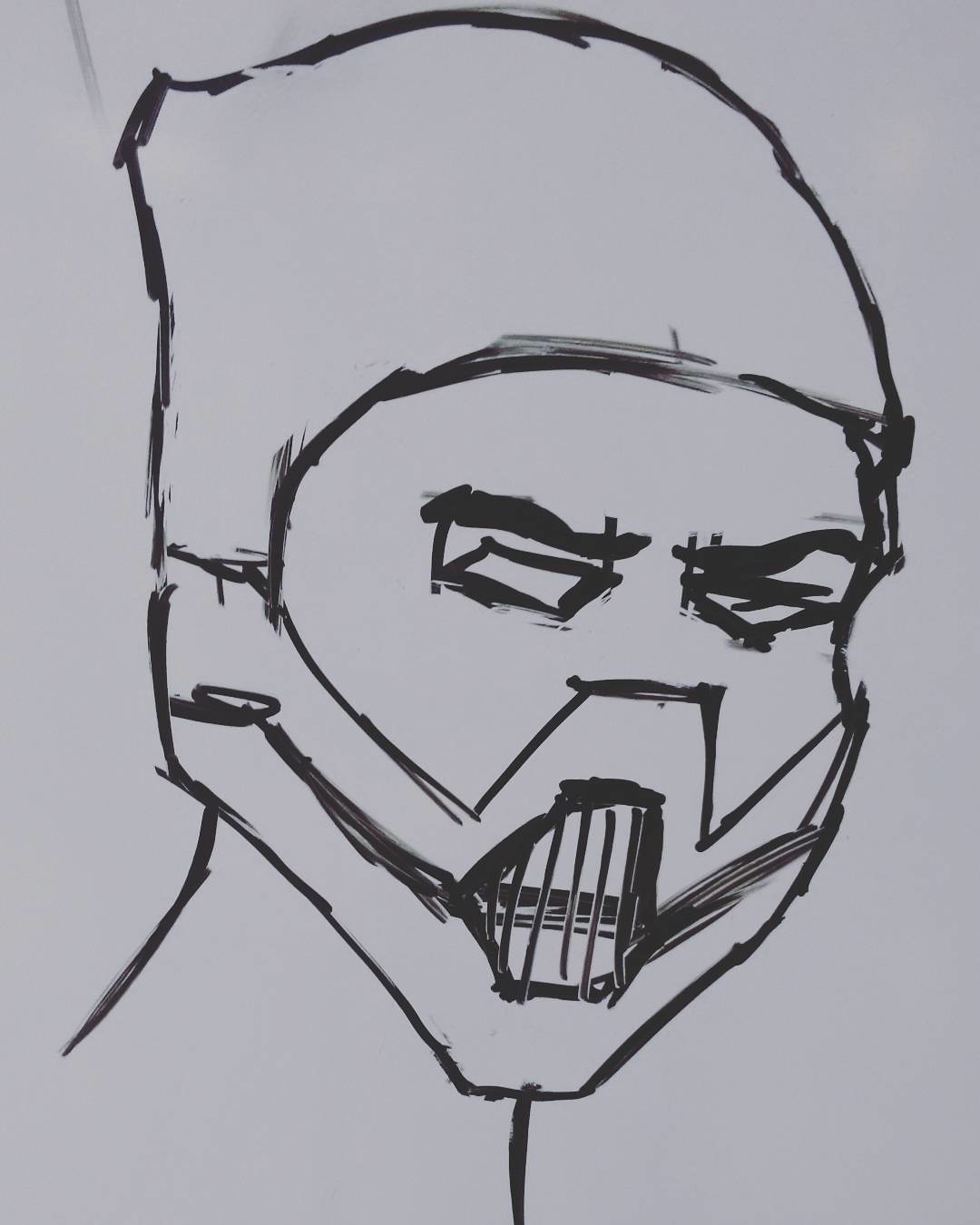This black and white image depicts a marker drawing of a character's face. The character is donning a hood, which creates a masked appearance. Notably, the eyes are square-shaped and lack pupils, adding to the eerie, mask-like feel. The face is covered by what resembles a grill-style Hannibal Lecter mask, contributing to a menacing aura. The character is depicted from the neck up, with visible portions of his neck. He is oriented slightly to the right, giving an impression of looking forward with a rightward bias. The drawing appears to be made with markers on a whiteboard, characterized by bold, unsophisticated lines, indicating a simplistic and rough art style.